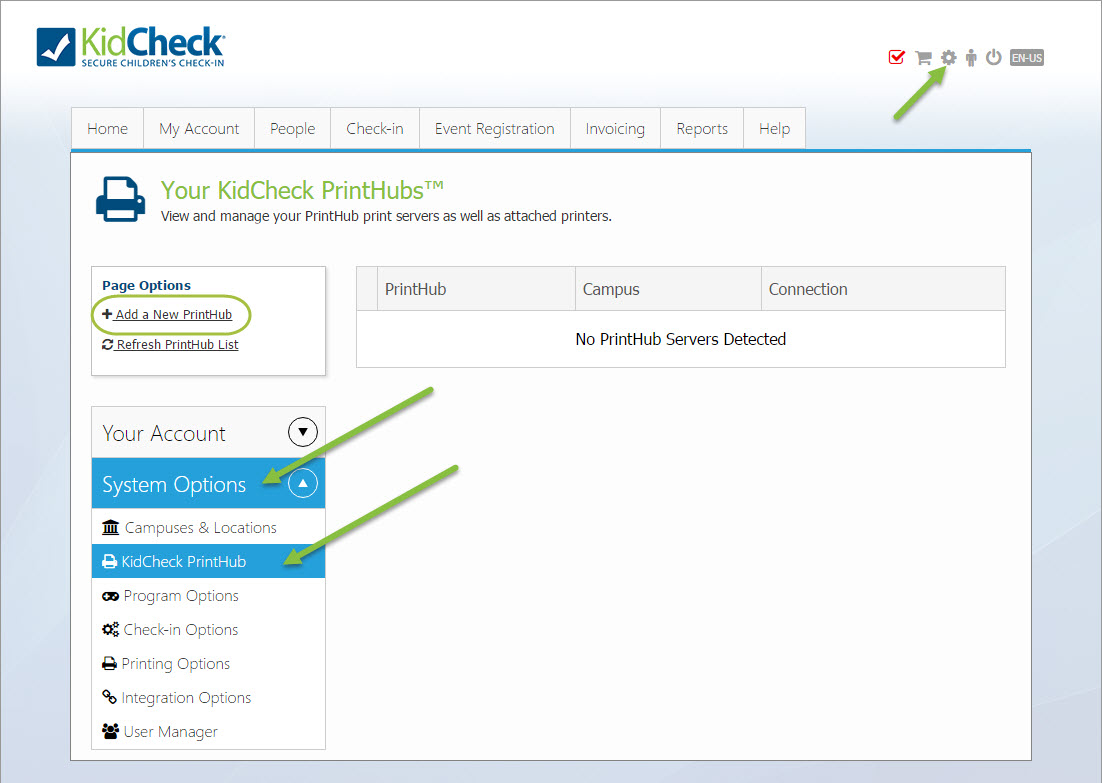This screenshot showcases the user interface of a Kid Check system aimed at secure children's check-in. The primary focus is a blue box with a checkmark icon and the text "Kid Check, Secure Children's Check-In," which is outlined in gray and exhibits various shades of blue within.

On the right side of the screen, icons for check, card, settings, person, power, and language (labeled as "English") are displayed, with a prominent green arrow pointing towards the settings icon.

Below this, a navigation menu appears with the following options: Home, My Account, People, Check-In, Event Registration, Invoicing, Reports, and Help, all set against a white background.

A section dedicated to printers is also visible, featuring an image of a printer and the heading "Your Kid Check Print Hubs, View and Manage Your Print Hub Print Servers, as well as Attached Printers." Options listed include "Page Options, Add a New Print Hub" (circled in green), and "Refresh the Print Hub." 

Towards the right-hand side, under "Print Hub, Campus Connection," a bold, black notice reads, "No Print Hub Servers Detected."

On the left-hand side, additional sections are detailed: "Your Account" and "System Options" (highlighted in a blue box with another green arrow). Further down, it lists "Campuses and Locations," followed by another blue box labeled "Kid Check Print Hub" with a green arrow. Finally, the menu includes "Program Options, Check-In Options, Printing Options, Integration Options, and User Manager."